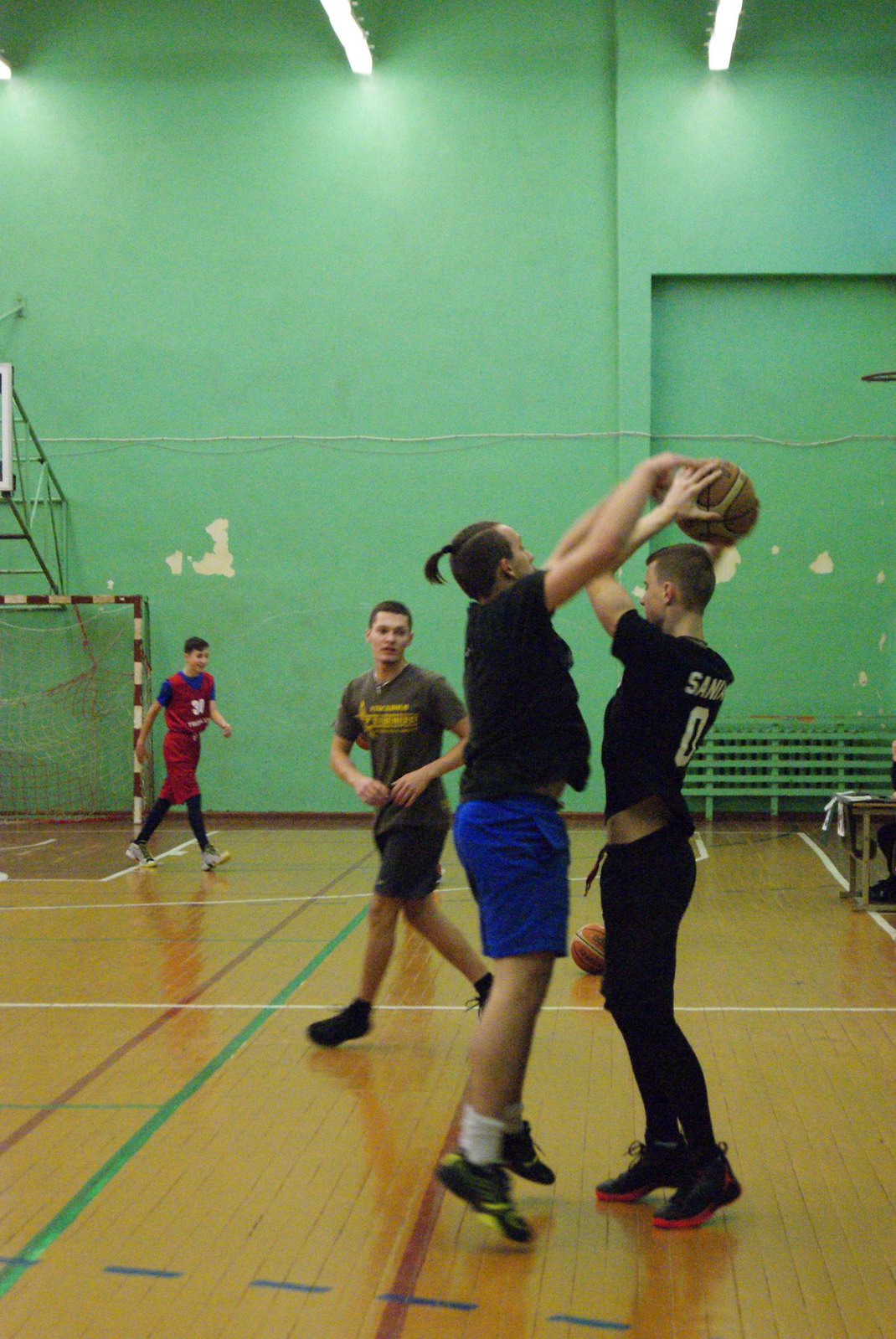Inside a school gymnasium, four men are captured engaging in a casual yet intense game of basketball. The gym has hardwood floors marked with green, red, and white stripes. The detailed setting reveals a green wall in the background with paint peeling off, exposing the underlying white plaster, and features a railing and indoor soccer goal posts.

Starting from the right side of the image, one man dressed in black sweatpants and a black t-shirt, partially revealing the number "0" and the letters "S-A-N" on it, is holding a basketball high in his hand, appearing ready to throw it. He stands sideways to the camera, with his stance exuding readiness and focus. He also sports black sneakers with red soles.

Next to him, leaping into the air is another man, who is trying to intercept the ball. He has a ponytail and is wearing a black t-shirt paired with blue shorts, complemented by black sneakers with yellow soles and white socks. His body language suggests a fierce determination to gain control of the ball.

In the background, a third man is visible, seemingly running. He is dressed in a green shirt with indiscernible text, dark shorts, and dark sneakers. His presence adds depth to the scene, emphasizing the ongoing motion and engagement of the players.

Further off in the distance, a younger individual, likely a teenager, is seen wearing a red top with "3-0" on it, red shorts, knee-length black stockings, and white sneakers. His positioning suggests that he is somewhat detached from the main action happening in the foreground.

Additionally, toward the middle right, there is a glimpse of a desk with someone seated behind it, partially visible through their knee, foot, and hand, adding a subtle yet realistic touch to the dynamic environment. On the middle left side, poles with a net strung between them can be seen, possibly indicating adjacent sports activities or equipment storage.

Together, these elements create a vivid, detailed snapshot of an indoor basketball game, rich with action and the texture of the gym’s setting.